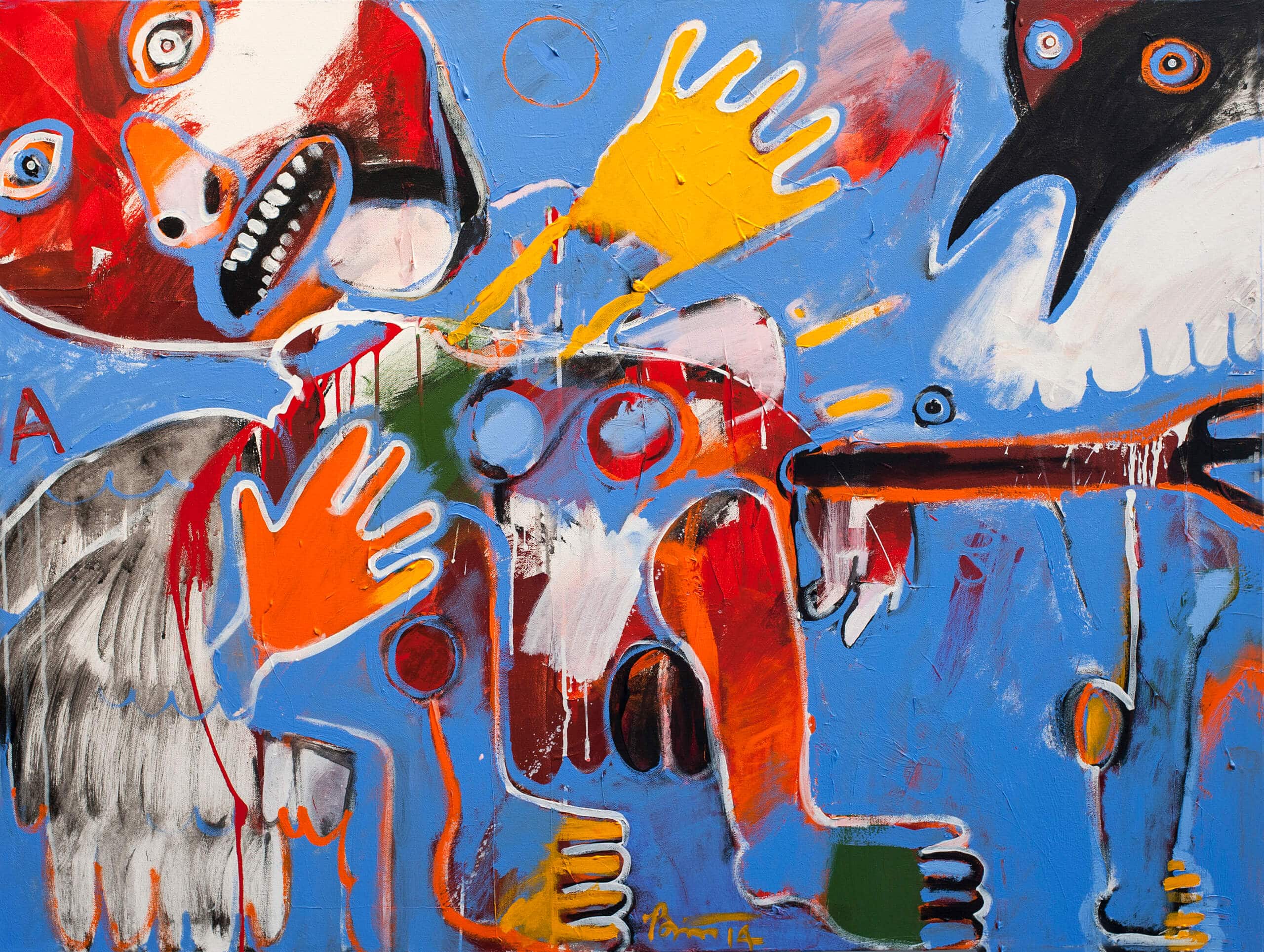This artistic piece is a vivid, abstract square painting without a border. The background features a painted blue wall, which sets the stage for an array of eclectic and surreal elements. In the center left, a bold red capital letter "A" stands out, anchored below by delicate white feathers, possibly representing bird wings. The upper left corner is dominated by an unsettling, multicolored human face with an open mouth, suggesting a scream, and mismatched eyes - one blue and one white. Nearby are two distinct handprints, one orange and one yellow. The composition also includes disjointed body parts; there are hand and leg elements, with legs painted blue and red. A strange, black creature with white wings and expressive blue eyes occupies the upper right corner, contributing to the eerie, dreamlike quality of the painting. This melding of human and animal forms, alongside vibrant and contrasting colors, creates a deeply abstract and surreal visual experience.